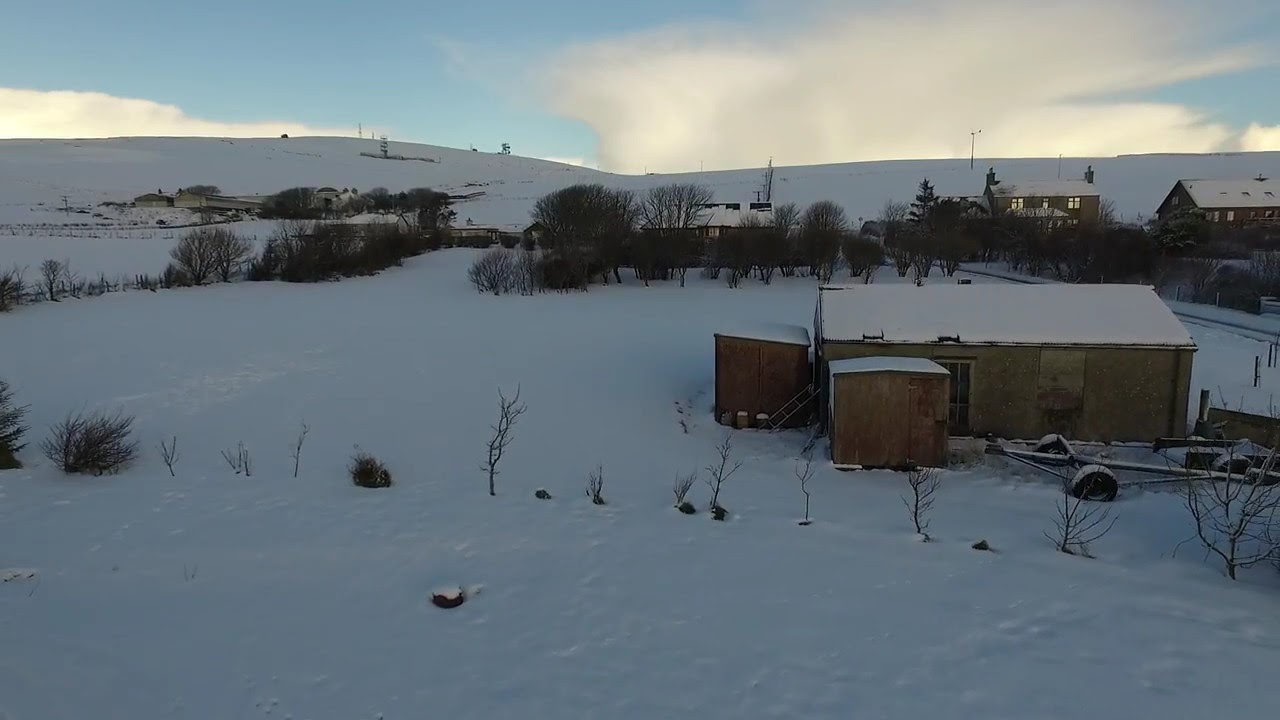This daytime photograph captures a rural, snow-covered hillside shrouded in shadows, contrasting sharply with a bright blue skyline adorned with stark white clouds, indicating sunlight from behind. The top quarter of the image features these luminous clouds, while the rest foregrounds a snowy, shaded landscape. Three houses are aligned on the hill, with the rightmost resembling a primitive, wooden shed or shack. There's an old barn or storage building towards the lower right corner, characterized by its squat, square form and rough exterior. A row of leafless trees and bushes stretches from the lower right to the left, framing the scene and reinforcing the winter atmosphere. In the upper left, a series of farm buildings lines the hillside, hinting at a sprawling ranch obscured by snow. The dominant colors are white from the pervasive snow, juxtaposed with blue sky and brown wooden structures.